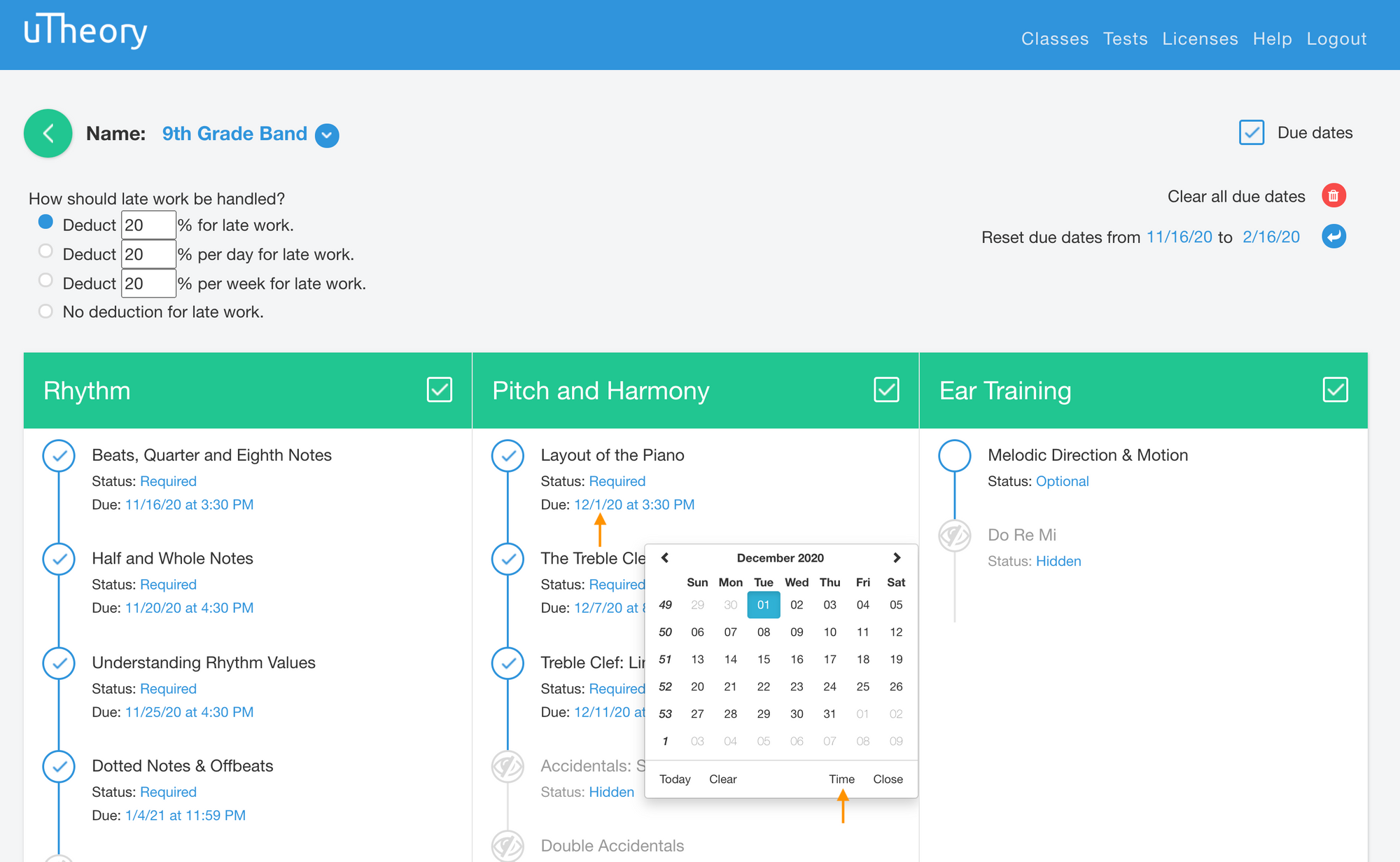This is a detailed screenshot of a webpage for "uTheory," framed within a blue border. At the top, there are several navigation tabs labeled "Classes," "Tests," "Licenses," "Help," and "Logout." Below this, a gray area features a green circle containing a white left-facing arrow. It displays information like the user's name, grade (ninth grade), and band, with this text being white. A blue circle with a white checkmark is also present.

Underneath, a prompt asks, "How should late work be handled?" Four options are listed, each within a bubble. The selected option, highlighted in blue, is "Deduct 20% for late work." Other options include "Deduct 20% per day for late work," "Deduct 20% per week for late work," and "No deduction for late work."

To the right, a box is marked with a blue check and labeled "Due Dates." Additional options below include "Clear all due dates" and "Reset due dates from 11-16-20 to 2-16-20," accompanied by a white left-facing arrow within a blue box.

The lower section of the page is green and divided into three categories: "Rhythm," "Pitch and Harmony," and "Ear Training." Each category features vertical entries. Under "Rhythm," the entries are "Beats, Quarters, and Eighth Notes," "Half and Whole Notes," "Understanding Rhythm Values," and "Dotted Notes and Offbeats." The "Pitch and Harmony" section includes "Layout of the Piano," an unreadable entry due to an overlaid calendar, "The Treble Clef," and more. The "Ear Training" section lists "Melodic Direction and Motion."